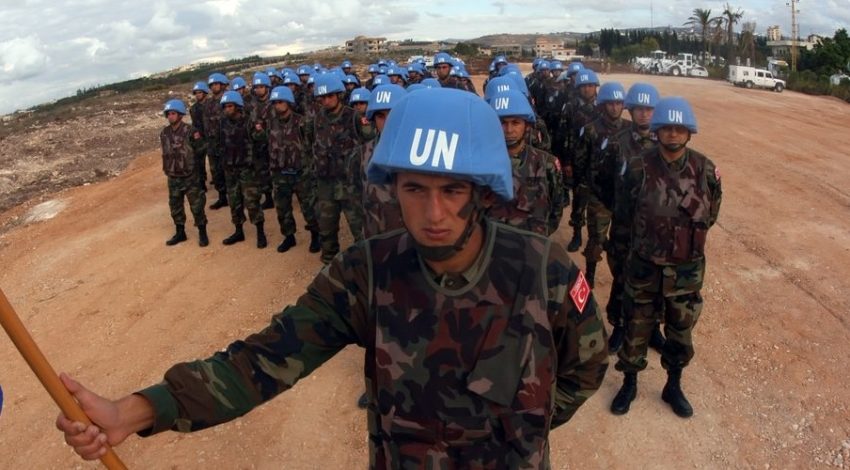This image shows a disciplined formation of over 20 UN soldiers, all sporting camouflage fatigues in shades of green, black, and brown, complemented by their distinctive blue helmets emblazoned with the white "UN" text. The troops, who appear to have brown skin, are lined up in roughly eight rows, adopting a square formation, with hands uniformly placed behind their backs. At the forefront, a leading soldier holds a pole, presumably a flag. The setting appears to be a dirt road with a red, sandy surface, possibly located in Africa or the Middle East. The background features white trucks, palm trees, various buildings, and scattered rocks and debris. The sky is blue with some clouds, highlighting the daytime atmosphere. A red badge is noticeable on the left shoulders of the soldiers' uniforms, adding a touch of uniformity and distinction to their appearance. The overall mood is somber and serious, reflecting the soldiers' focused demeanor.